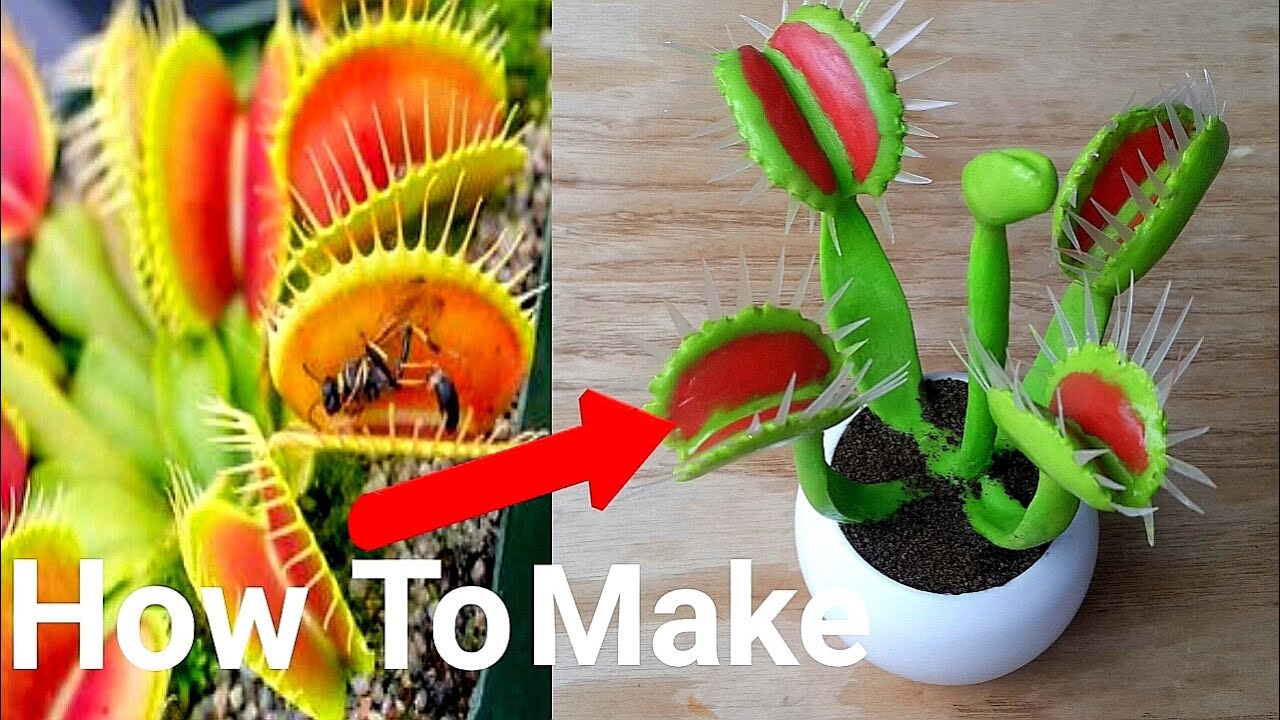This composite photograph comprises two images placed side by side, with a prominent red arrow pointing from the left image to the right image. Spanning across both images at the bottom, in large white text, are the words "how to make." The left image showcases an actual Venus flytrap, its green leaves blurred in the background. The jaws of the flytrap are a striking yellow with red interiors, and one of the jaws appears to trap a bee. The right image features a sculpted version of a Venus flytrap, meticulously crafted from green clay with vibrant red interiors and foil-like teeth. This sculpted plant, consisting of four flytrap heads around a central stalk with a bud, is placed in a white vase filled with black soil. The detailed craftsmanship highlights how one might create a realistic-looking Venus flytrap from simple materials, illustrating the transition from natural to handmade through the visual cue of the red arrow.